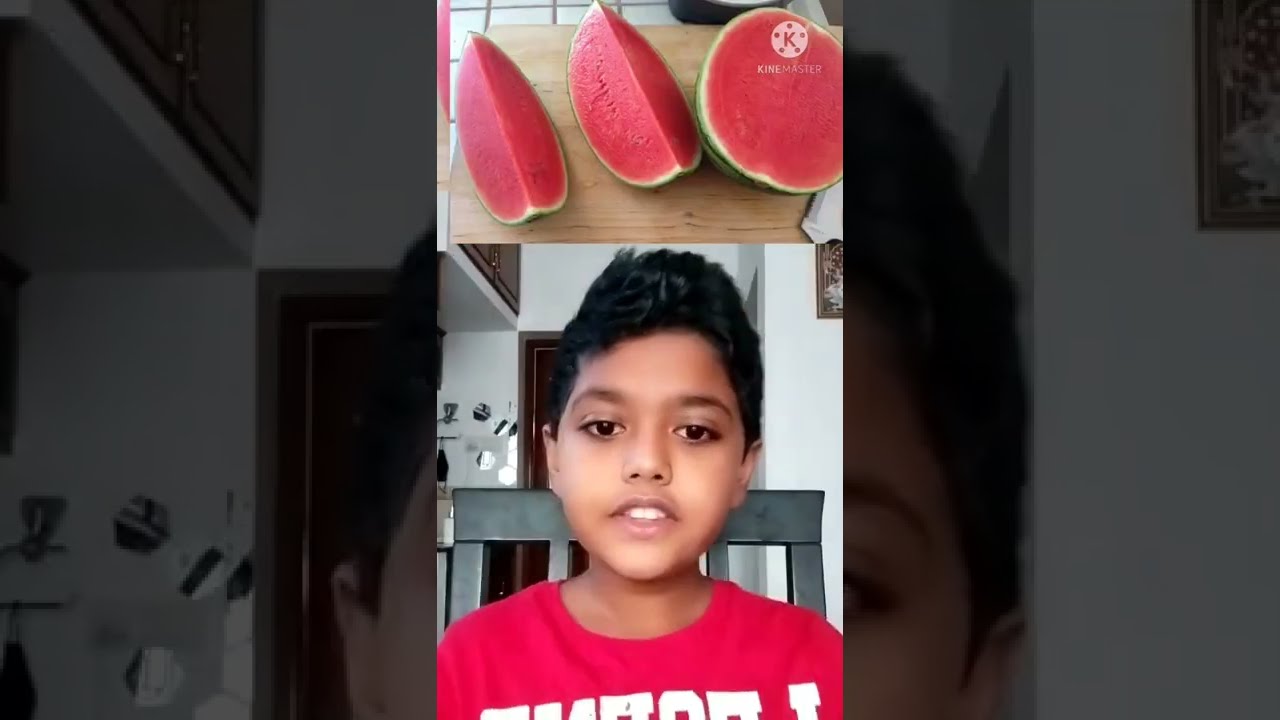This vertical photo captures a young Indian boy sitting in a dark gray or black chair against a backdrop of white walls. His spiky black hair and dark eyes draw attention, with his mouth open, revealing his teeth, as if he is speaking or about to present something. He is wearing a red t-shirt with white lettering. The sides of the image are darkened with a film-like effect, framing the central scene. 

Above the boy, a wooden cutting board with the inscription "Pink Master" prominently displayed bears a sliced watermelon: one half intact and the other half cut into quarters lengthwise. The boy's direct gaze into the camera suggests he might be preparing for a live stream, a presentation, or perhaps a playful skit. The overall ambiance suggests a casual, home environment with the boy set against the stark contrast of the dark sides, adding a cinematic touch to the moment.